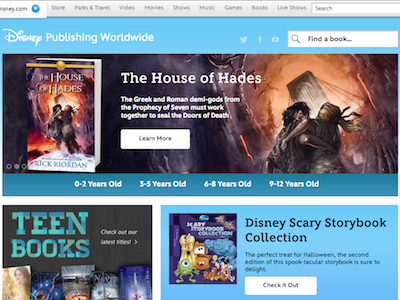The image captures a screenshot of a Disney.com webpage displayed on a computer or mobile device. At the very top of the webpage, a navigation bar is visible with clickable links for various sections: store, parks and travel, video, movies, shows, music, games, books, and live shows. A search bar is also prominently featured on this navigation row.

Beneath the navigation bar, the page is titled "Disney Publishing Worldwide." To the right-hand side, icons for Twitter, Facebook, and YouTube are displayed, suggesting options for social media engagement. 

Further down the page is another search bar labeled "Find a book..." Alongside this, the focal point of the screenshot is an advertisement for a book titled "The House of Hades" by Rick Riordan. The book cover illustration depicts two eerie figures navigating through a sinister-looking house. Accompanying text states: "The Greek and Roman demigods from the Prophecy of Seven must work together to seal the doors of death," and a "Learn More" button allows for further exploration.

Additional sections on the page categorize book recommendations by age groups: zero to two-year-olds, three to five-year-olds, six to eight-year-olds, and nine to twelve-year-olds.